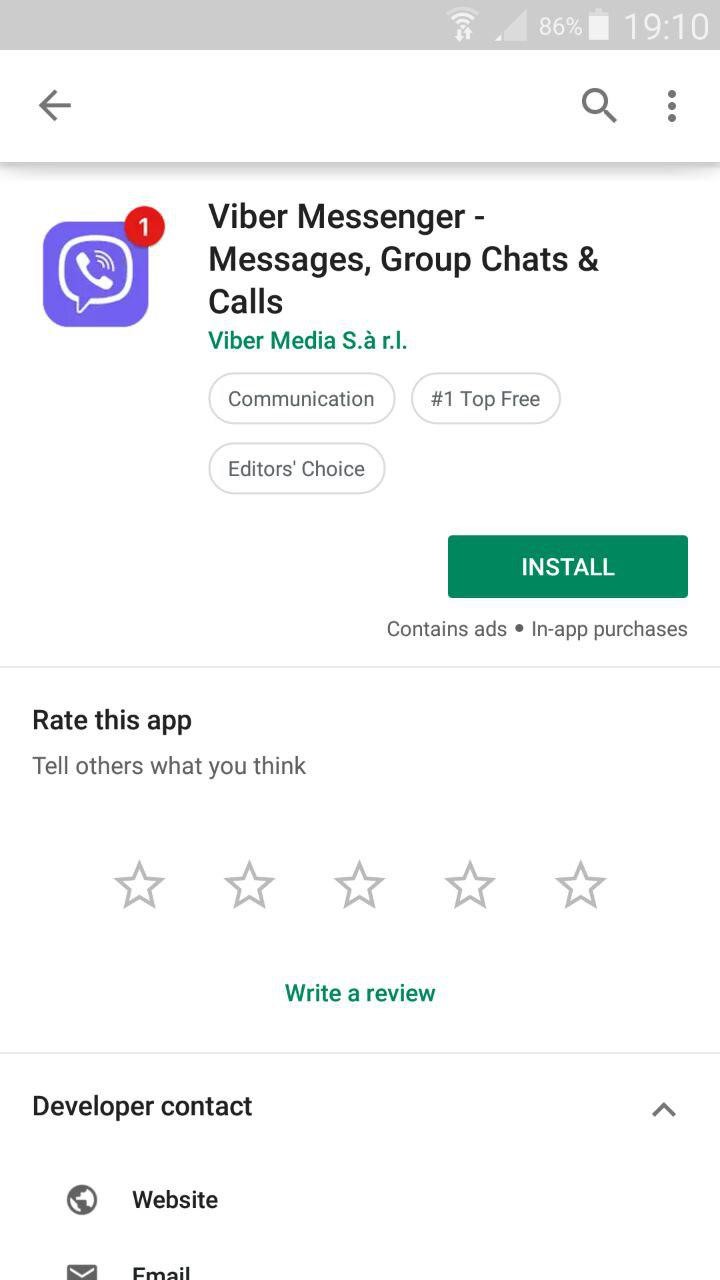The webpage features a dark grey bezel at the top. On the right-hand side, there is a wireless signal icon with three out of four bars highlighted. Adjacent to it is a cellular signal icon which is nearly at the bottom, accompanied by an 86% battery indicator. Displayed next is the time set to 1910 in military format.

Below the bezel is a white rectangle. On its left side, there is a black arrow, while the right side features a magnifying glass icon and three ellipses for settings. Directly underneath this section, there is a purple square with a rounded white inner square depicting a landline phone emitting three bent lines of increasing size, indicating sound or notification. This icon is accompanied by a red circle with a white numeral one inside it.

Next to this icon, the text "Viber Messenger - messages, group chats, and calls" is written in red. Beneath this, in green text, it says "Viber Media S.A. R.L." with accent marks. Further down, there is a white oval labeled "Communication" written in black. Adjacent to it is another oval denoting "No.1 Top Free" and an oval labeled "Editor's Choice." On the right-hand side, a dark green rectangle contains white text that reads "Install."

Below this, in black text, it states "Contains Ads" followed by a dot, and then "In-App Purchases." Further down, it invites users to "Rate This App, Tell Others What You Think," with a 0 out of 5 stars rating shown and the option to "Write a Review" in green.

Further options include a contact section with an upward-pointing arrow. There is a globe symbol next to the text "Website," followed by an envelope icon indicating email.